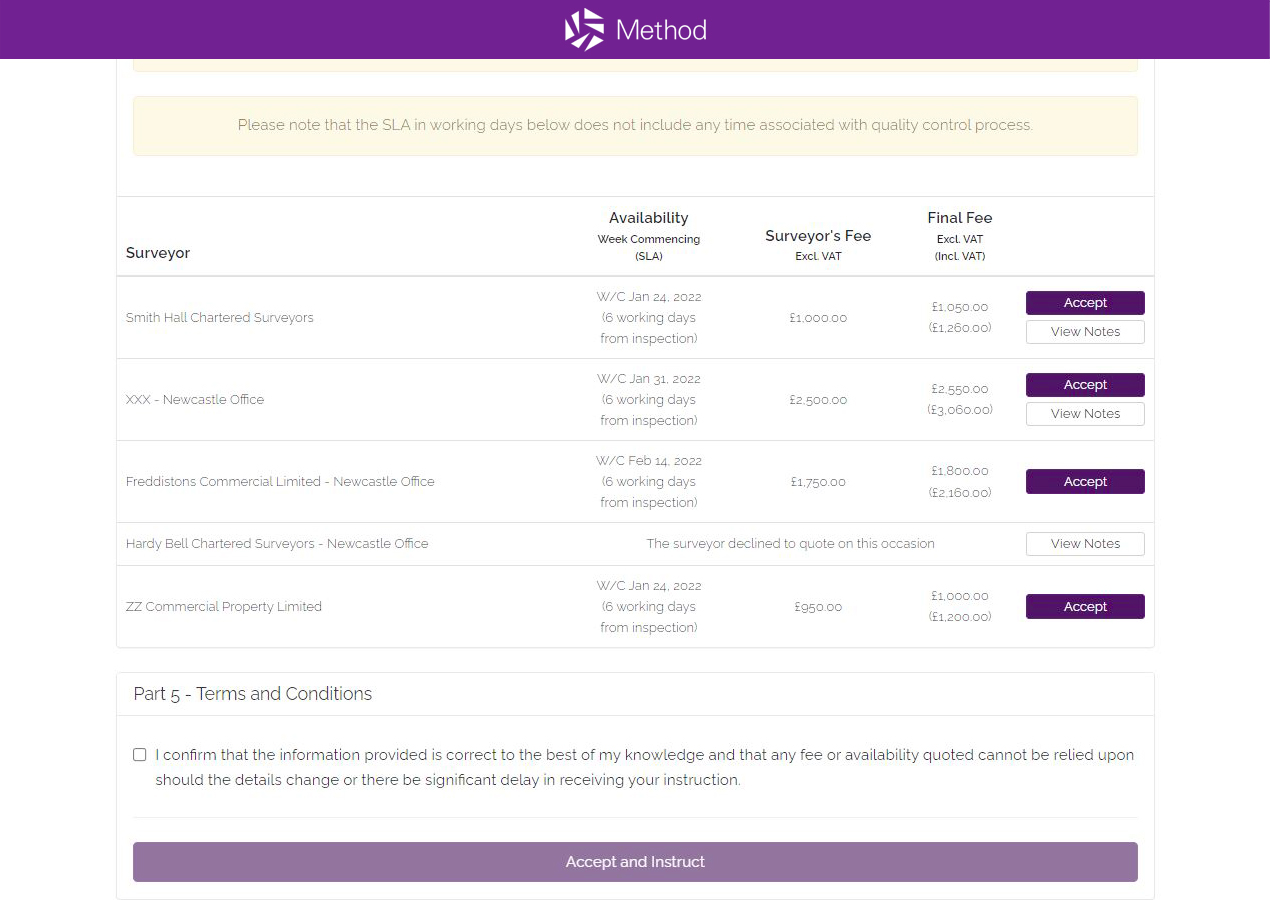In the image, the top section features a large purple box labeled "Method," adorned with a set of small white triangles arranged to almost form a circle. Below this, a search box is situated, followed by text that reads "Surveyor," "Availability," "Surveyor's Fee," and "Final Fee." The print beneath these headers is quite small and blurry. On the right side of the image, there are several purple "Accept" buttons and white "View Notes" buttons corresponding to a list of four items. Towards the bottom, the image includes section titled "Part Five Terms and Conditions," accompanied by a checkbox with the statement: "I confirm that the information provided is correct to the best of my knowledge, and that any fee or availability quoted cannot be relied upon should the details change or there be significant delay in receiving your instruction." Finally, a large purple box at the very bottom contains the text "Accept and Instruct Only."